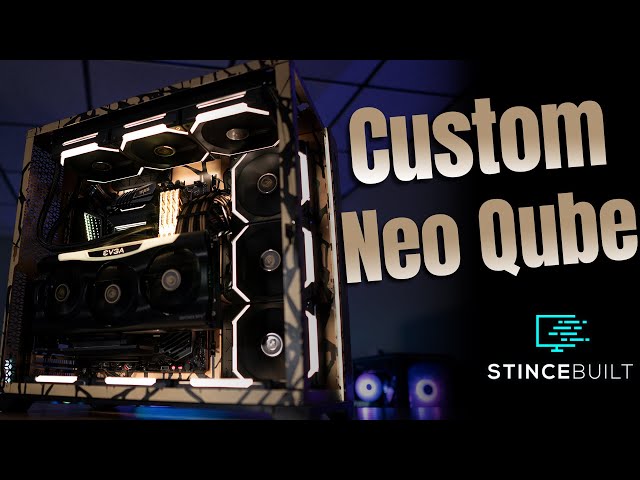The image is a rectangular advertisement for a custom-built computer, surrounded by thin black borders on the top and bottom. The left side of the image features a photograph of a large, sleek computer tower. The tower has three see-through sides made from brownish acrylic plastic, showcasing its intricate internal components. Prominently visible inside the tower are multiple cooling fans arranged both horizontally at the top and vertically along the side. The computer is equipped with an EVGA graphics card that features three additional cooling fans. The illuminated interior, with strategically placed lighting around the fans and the bottom, highlights the motherboard and complex wiring.

To the right of the computer tower, in gold and white block text against a dark navy blue background with black accents, the advertisement reads "Custom Neo Cube." Below this, it states "Since Built," accompanied by a blue logo resembling a screen with lines. This striking image, possibly a screen capture from a YouTube video or thumbnail, captures the sophisticated and high-performance nature of the custom-built Neo Cube PC.